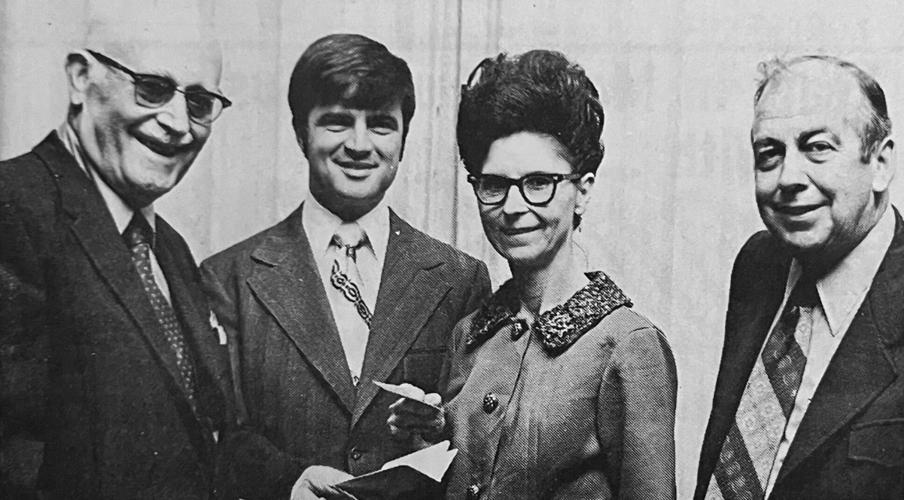This black-and-white photograph, likely taken in the 1940s or 1950s, features a group of four Caucasian individuals — three men and one woman — standing in front of a light gray wall. The image is horizontal and rectangular, capturing them from mid-torso up. The men are all dressed in dark suits with ties over button-down shirts, embodying the formal style of the time.

On the far left is an older, bald man wearing black-rimmed glasses, a dark suit, and a spotted tie. He sports a friendly smile. Next to him stands a younger man with full, dark (possibly black) hair, dressed in a dark suit and a white button-down shirt. He is holding some papers and also smiles warmly at the camera.

The woman is positioned in the middle, slightly to the right. She wears a long-sleeved dress or button-up blazer adorned with large buttons and a prominent floral collar. Her hair is styled in a beehive, and she wears dark-rimmed glasses. She appears to be receiving a card or brochure from the man next to her.

On the far right is another older man with a receding hairline. He wears glasses similar to the first man’s, along with a dark suit and a tie over a white button-down shirt. He, too, smiles at the camera, contributing to the friendly and formal atmosphere of the photograph.